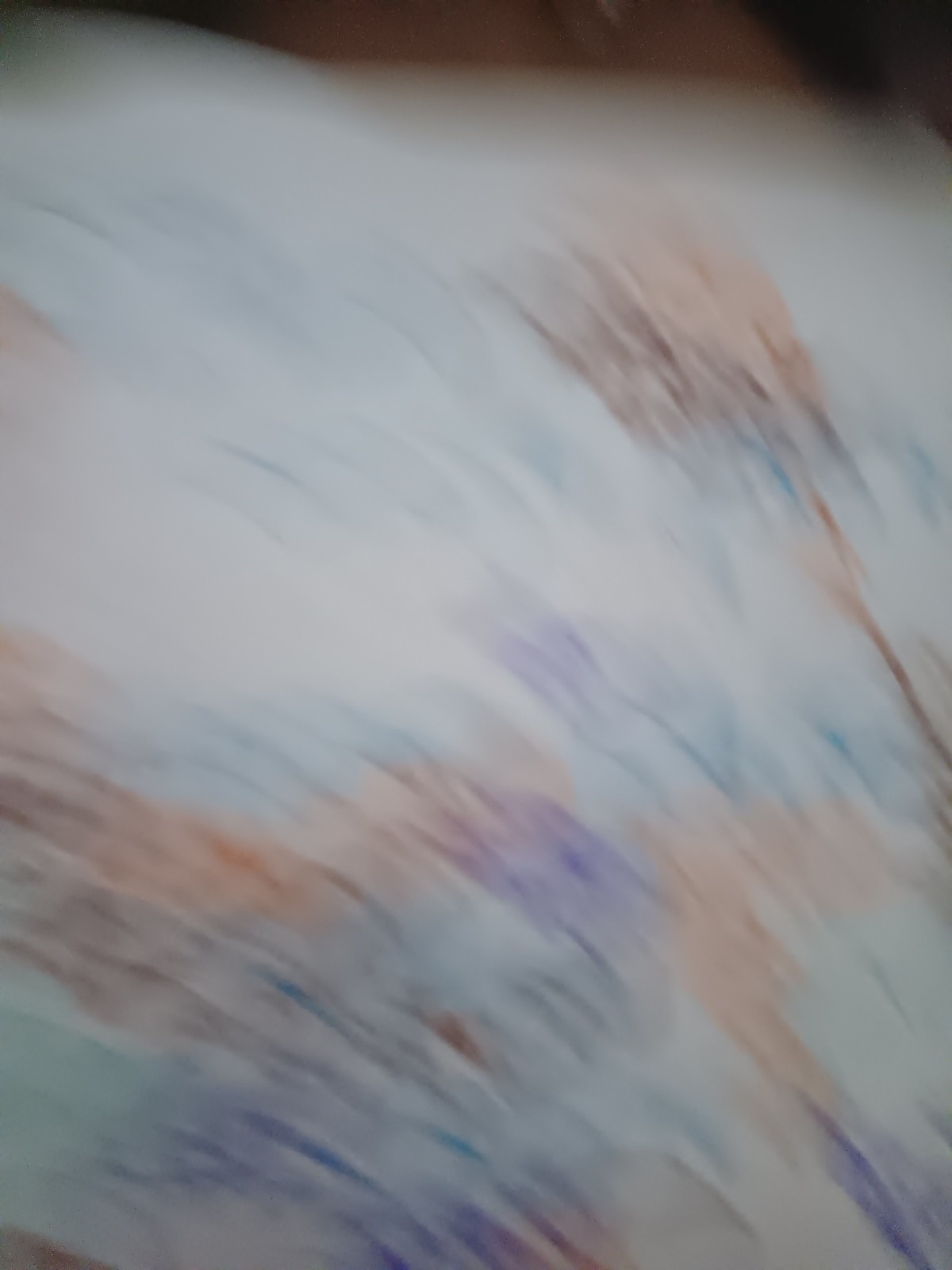A highly blurred image depicting what seems to be either a watercolor painting or a child's rudimentary drawing. The motion-blurred photograph makes it difficult to discern specific details, but prominent light orange and blue hues are visible against a white or off-white background. Amid the color streaks, there appears to be an attempt at portraying a tree, though the blurriness renders it indistinct and abstract. The photo's overall disorienting effect leaves it open to interpretation, with objects melding into amorphous shapes and colors.